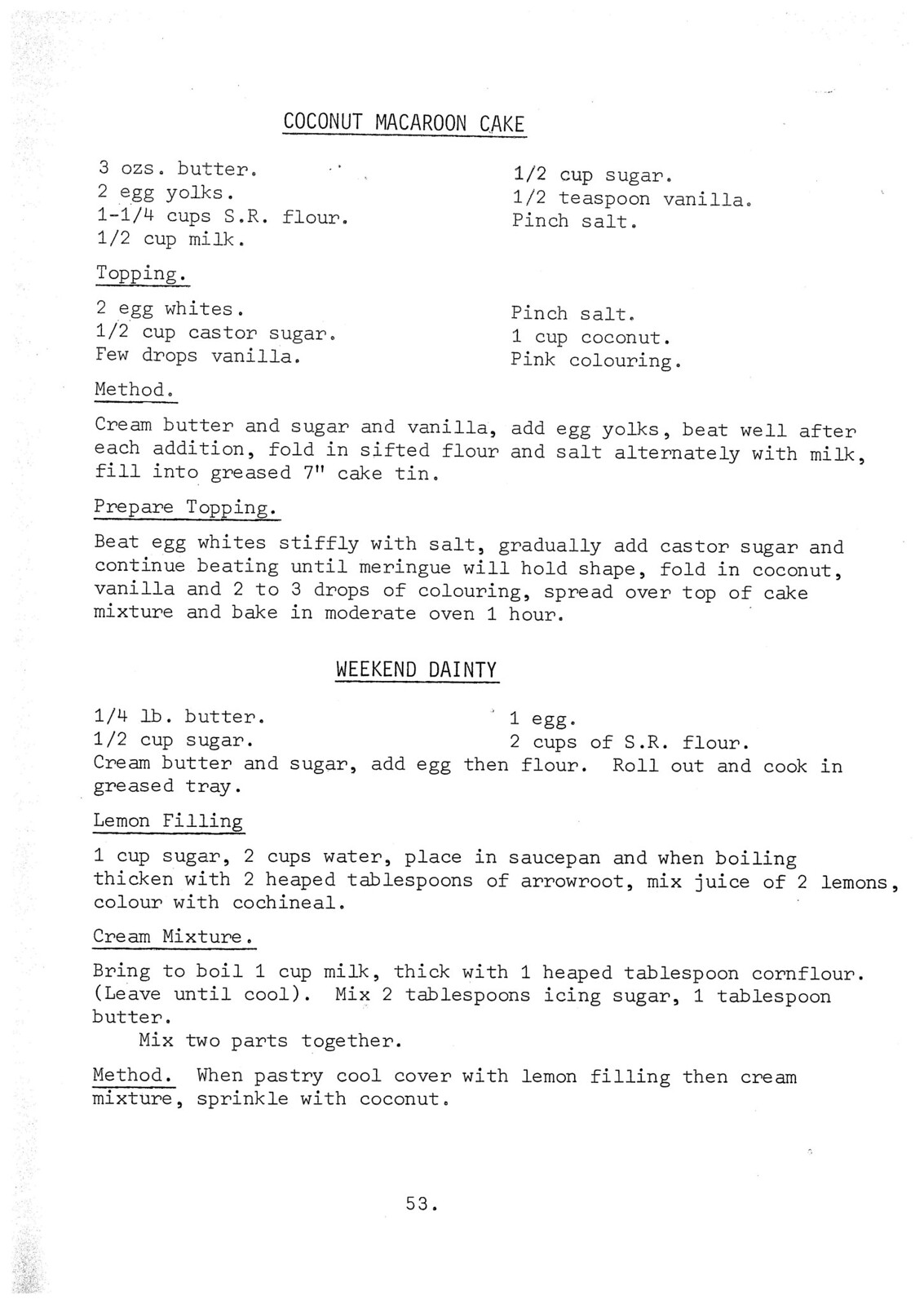The image depicts a white page numbered 53 containing two typed recipes: Coconut Macaroon Cake and Weekend Dainty. The Coconut Macaroon Cake recipe lists the following ingredients: 3 ounces of butter, 2 egg yolks, 1 1⁄4 cups of self-raising flour, 1 1⁄2 cups of milk, 1 1⁄2 cups of sugar, 1 1⁄2 teaspoon of vanilla, and a pinch of salt. For the topping, the ingredients are 2 egg whites, 1 1⁄2 cups of caster sugar, a few drops of vanilla, a pinch of salt, 1 cup of coconut, and pink coloring. The method instructs to cream the butter, sugar, and vanilla, add egg yolks and beat well after each addition, then fold in sifted flour and salt alternately with milk. The mixture is to be poured into a greased 7-inch cake tin. For the topping, beat the egg whites stiffly with salt, gradually add caster sugar while continuing to beat until the meringue holds its shape, then fold in the coconut, vanilla, and 2-3 drops of coloring. Spread the topping over the cake mixture and bake in a moderate oven for one hour.

The second recipe, Weekend Dainty, requires 1/4 pound of butter, 1 egg, 1/2 cup of sugar, and 2 cups of self-raising flour. The directions are to cream the butter and sugar, add the egg, then mix in the flour, roll out the dough, and cook on a greased tray. The lemon filling consists of 1 cup of sugar and 2 cups of water, boiled and thickened with 2 heaped tablespoons of arrowroot, then mixed with the juice of 2 lemons and colored with cochineal. For the cream mixture, bring 1 cup of milk to boil, thickened with 1 heaped tablespoon of corn flour, and let it cool. Mix in 2 tablespoons of icing sugar and 1 tablespoon of butter, then combine this mixture with the lemon filling. When the pastry cools, cover it with the lemon filling and then the cream mixture, and sprinkle with coconut.